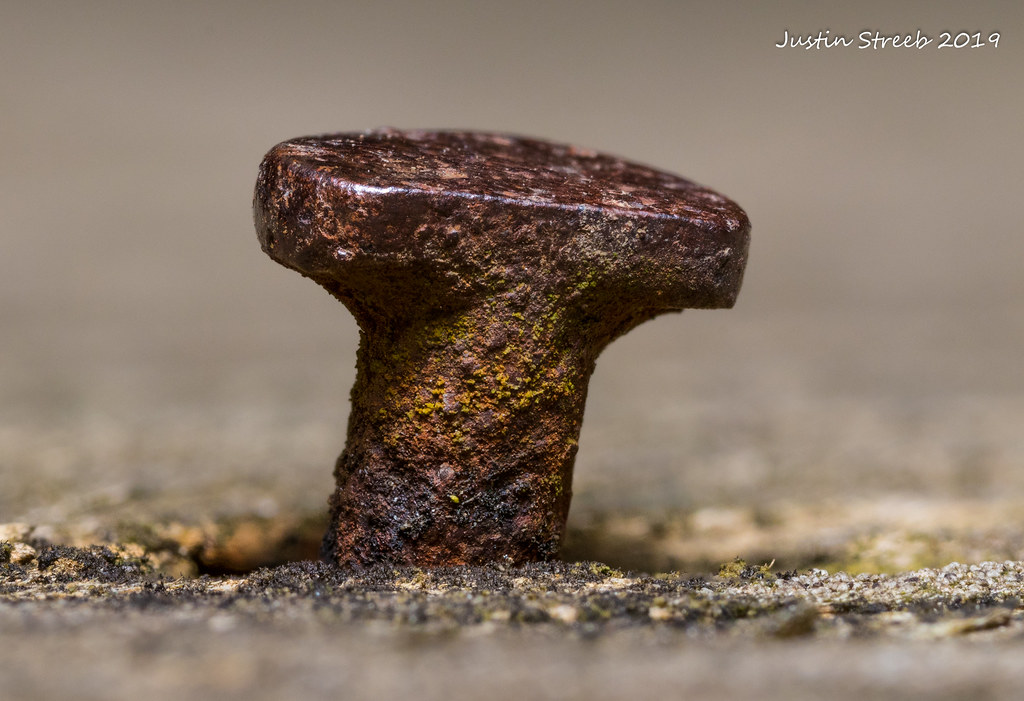This close-up photo captures a highly corroded piece of metal, possibly the head of an old nail, seen from a side profile. The metal object is shaped like an uppercase T, with a wide base and a relatively short top section. It's completely covered in rust, featuring jagged and sharp surfaces. The corrosion creates a gradient of colors: black and red at the bottom where it meets a black and beige gritty ground, transitioning to shades of yellow, brown, and black as you move upwards, and finally, to a rust-colored and slightly shiny head. The background is a blurred beige or gray, emphasizing the texture of the metal. In the upper right corner, the image is signed in white text: "Justin Streeb, 2019."